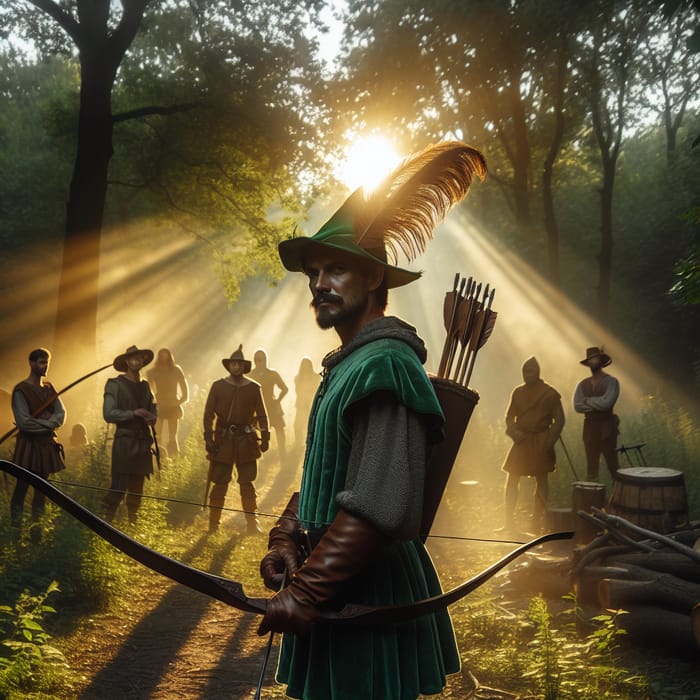The image depicts a realistic rendering of a character resembling Robin Hood, standing in a forested area. The man, sporting a mustache and goatee, has a determined and stern look on his face. He wears a pointy green velvet hat adorned with a large brown feather that extends upward and to the right. His attire includes a light and dark green suit, gray sleeves, and dark brown leather gloves that reach up to his elbows. Slung across his back is a quiver filled with wooden arrows, and he holds a dark brown recurve bow with a black string at his waist, with an arrow nocked and his hand resting on it.

Behind him, a row of eight men stand, some with folded arms and others with their hands by their sides. They are similarly dressed, though only Robin Hood has the distinctive feathered hat. Sunlight streams through the tall green trees in the background, casting an orange glow on the group. To the right, partially obscured by the men and trees, is a whiskey barrel standing upright with a rounded top and a few logs and barrels scattered nearby. The illustration melds realistic elements with a fantasy aesthetic, capturing the essence of a legendary archer and his band of followers in a serene, sunlit forest.